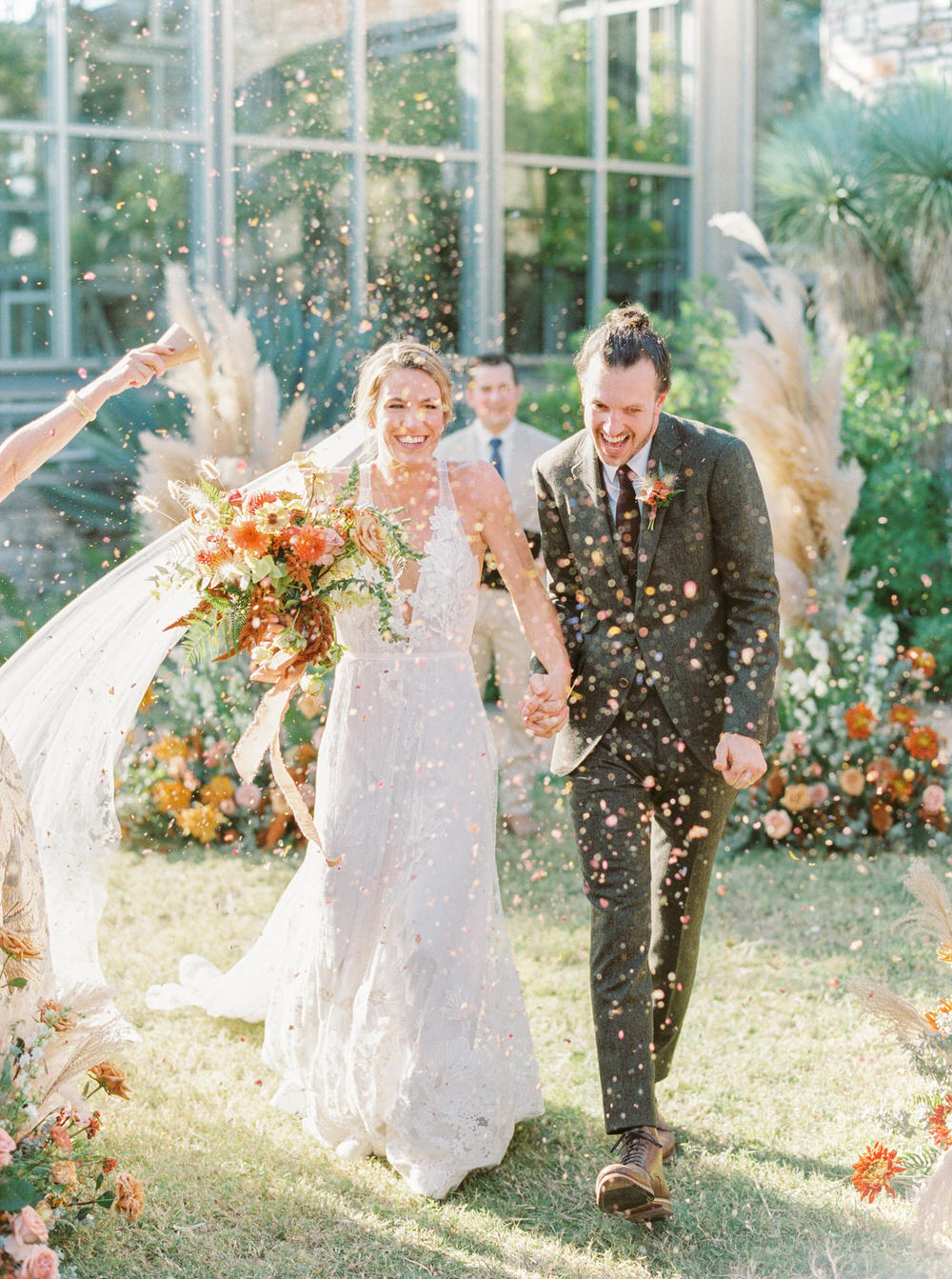In the bright midday sun, a newlywed couple walks forward through a shower of confetti during their outdoor wedding celebration. The bride, positioned on the left, is Caucasian with blonde hair parted to the side and pulled back, a bridal veil gently floating to the left. She wears a sleeveless white halter dress with a low v-neckline extending to the waist, and carries a bouquet featuring yellow and orange flowers accented by green fern leaves in her right hand, while holding her groom's hand with her left. The groom, also Caucasian, stands to her right, wearing a dark gray suit paired with a brown tie and brown shoes. He has a neatly trimmed beard and his dark brown hair is styled in a man bun. A boutonniere matching the bride's bouquet decorates his lapel. Both are beaming with joy, the groom's smile open and bright.

Behind them, slightly out of focus, stands the officiant, a Caucasian man wearing a light tan suit with a blue tie, holding what appears to be a Bible. Large, wild pampas grass and various flower arrangements flank the couple on either side, adding a natural touch to the scene. The wedding takes place on a verdant lawn, framed by a large building with many windows in the background. Numerous hands, including a visible arm on the left, are tossing confetti, enveloping the couple in a celebratory cloud. The carefree ambiance, coupled with the radiant sunlight streaming from the left, highlights the joy and love of this significant moment.